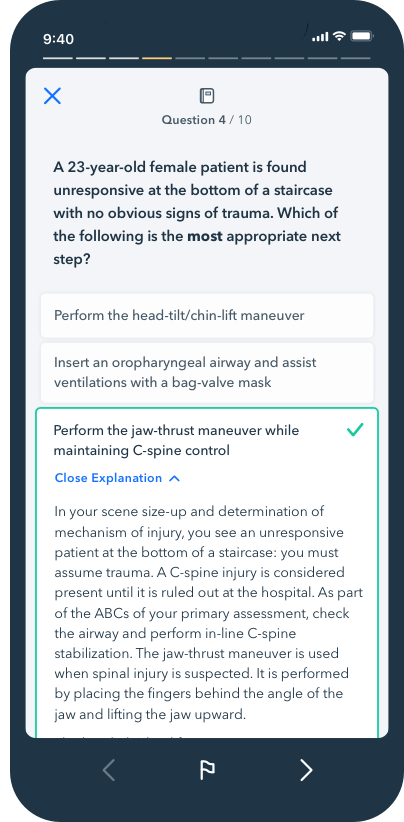The image depicts a black cell phone screen turned face up. At the top of the screen, the time reads 9:40, and it shows full network coverage, Wi-Fi connectivity, and a fully charged battery. Below this, an icon resembling a book is displayed, with the text "Question 4/10" beneath it.

The question presented on the screen reads: "A 23-year-old female patient is found unresponsive at the bottom of a staircase with no obvious signs of trauma. Which of the following is the most appropriate next step? Perform the head tilt/chin lift maneuver. Insert an oropharyngeal airway and assist ventilations with a bag valve mask. Perform the jaw thrust maneuver while maintaining C-spine control." The third option, "Perform the jaw thrust maneuver while maintaining C-spine control," is highlighted in green and marked with a green check mark.

An explanation follows: "In your scene size-up and determination of the mechanism of injury, you observe an unresponsive patient at the bottom of a staircase. You must assume trauma. A C-spine injury is considered present until it is ruled out at the hospital. As part of the ABCs of your primary assessment, check the airway and perform inline C-spine stabilization. The jaw thrust maneuver is used when spinal injury is suspected. It is performed by placing the fingers behind the angle of the jaw and lifting the jaw upward."

The image contains no photographic elements, people, animals, plants, flowers, or trees; it solely features text displayed on the cell phone screen.